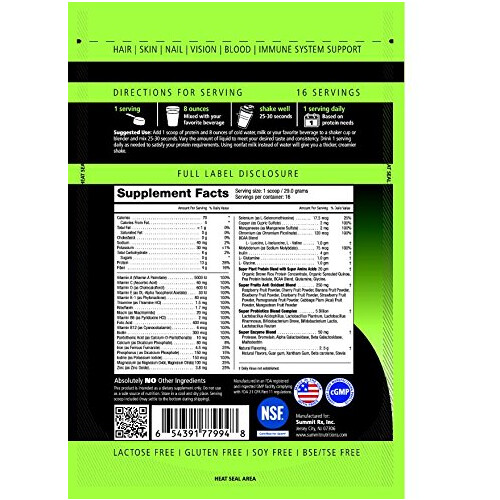The image is a detailed photograph of the backside of a nutritional supplement box, primarily in a neon green color. At the top, a green banner prominently displays the words "Hair, Skin, Nail, Vision, Blood, Immune System Support" in black text. Below this banner, on a black and green mixed background, are the "Directions for Serving," indicating there are 16 servings in total. The serving instructions, written in white text, include phrases like "one serving," "eight ounces," "shake well," and "one serving daily," though some text is too tiny to be easily readable. A neon green label underneath proclaims "Full Label Disclosure." Further down, a traditional white box with black text provides the "Supplement Facts," detailing the ingredients and nutritional information. Beneath this section, the label clearly states "Absolutely no other ingredients." At the bottom, it lists various product attributes, including "Lactose Free, Gluten Free, Soy Free, BSE/TSE Free." Additionally, there are a barcode, a square QR code, and some logos, including NSC and another unclear logo. The very bottom text, albeit very tiny, reads "Heat Seal Area."